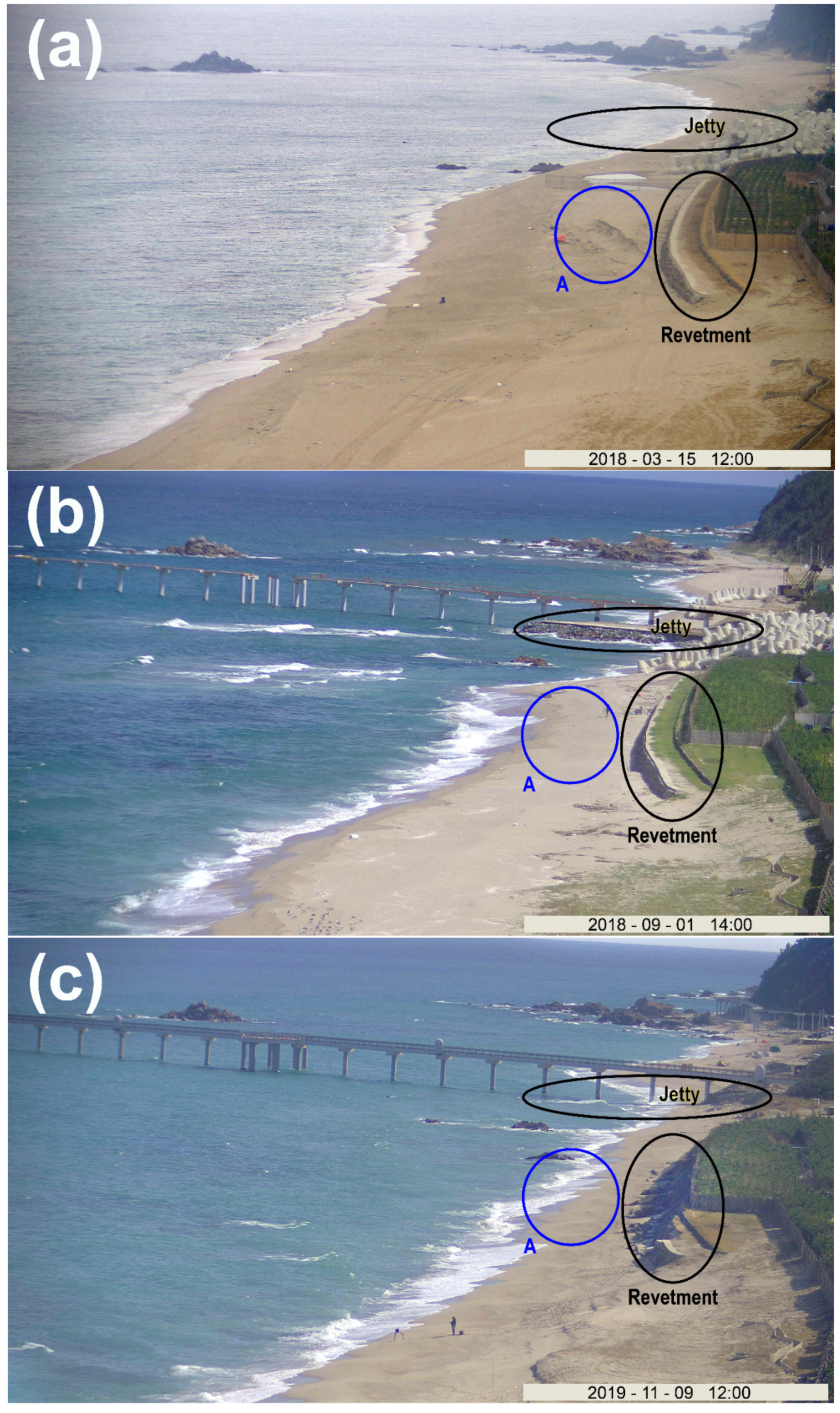The image displays a series of three stacked photographs labeled A, B, and C in white font at the top left corner of each image. Each photo captures a beach scene from a similar angle, highlighting changes over time. The top image (A) depicts a beach with a lot of sand and gray water, and it includes two ovals on the right side labeled "jetty" and "revetment," with a blue circle marking "A." Dates on these images are: A - March 15, 2018; B - September 1, 2018; C - November 9, 2019. Notably, images B and C, which feature bluer ocean water, green grass on the beach, and a pier, appear almost identical. In contrast, image A lacks the pier shown in the subsequent photos.